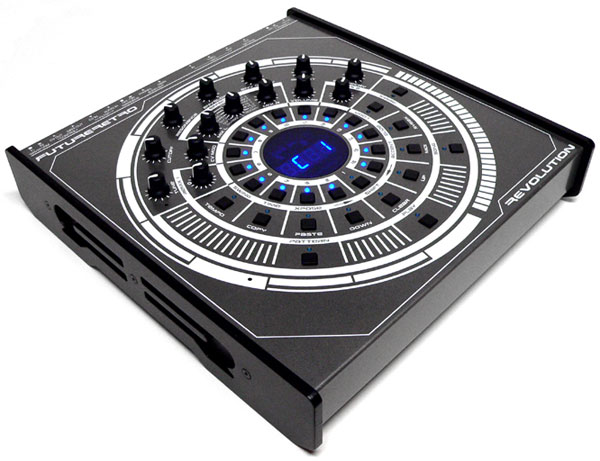This image is a color photograph of an electronic soundboard, set against a white background with no frame, signature, or date. The soundboard itself is square and composed of black metal, captured at an angle that makes the corners point up, down, and to the sides, rather than sitting flush within the photograph. The design of the soundboard features a series of white concentric circles that evoke the look of a vinyl record, with the center circle housing a blue digital display showing "C1." Surrounding this center display are numerous black knobs, each marked with a white line and oriented in various directions. Additionally, some control knobs are distributed along the top and left-hand side of the device. The upper left corner of the soundboard bears the partially legible label "Future Retro," and the bottom right corner displays the word "Revolution." Overall, this sophisticated piece of musical or DJ equipment integrates a variety of control functions, indicated by additional labels and markings, possibly related to tempo, copy, paste, down, clear, and up settings.